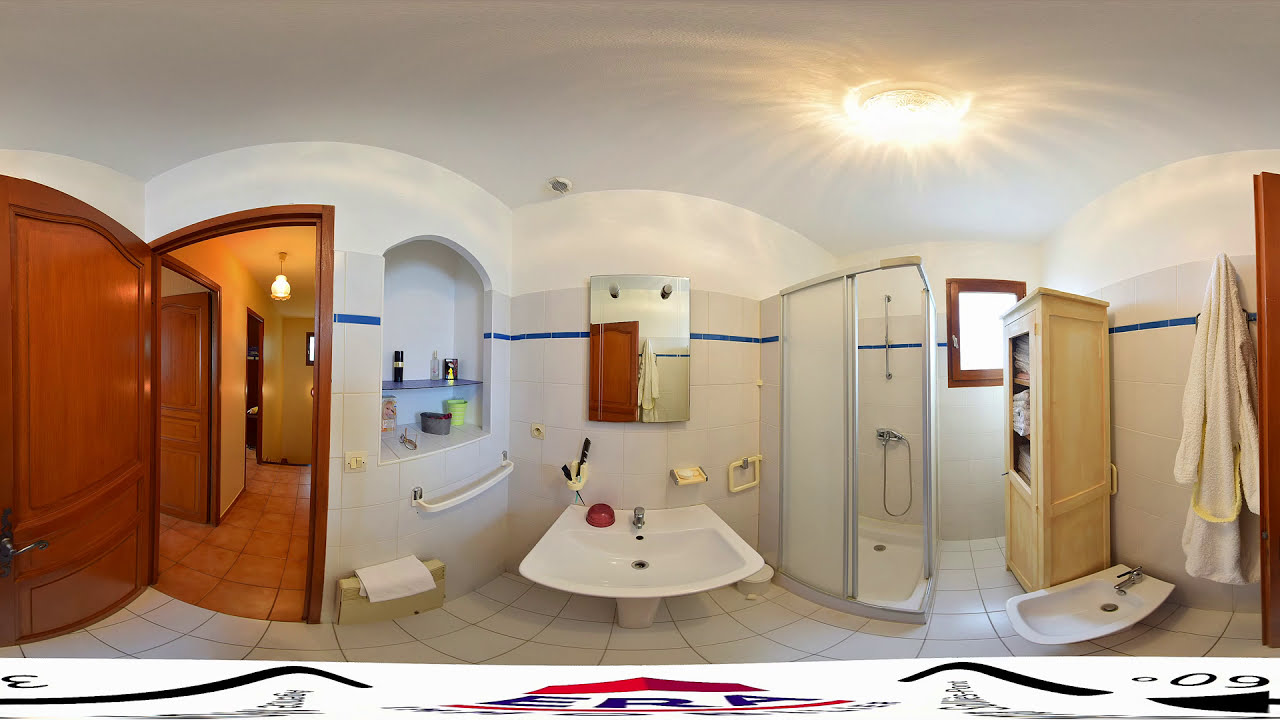This panoramic photograph provides a detailed view of a large bathroom. The bathroom features white walls and ceiling, complemented by white tile flooring interspersed with tiles that have small blue stripes. Centrally positioned in the photograph is a sink with a mirror above it. To the left of the sink and mirror, a built-in shelving unit holds various items, including a pair of glasses, a box of hair dye, a lime green pot, and a dark grey basket on one shelf, with three bottles of perfume on a higher shelf. Additionally, there is a holder containing a toothbrush, a hairbrush, and an eyebrow brush, and an empty towel rail nearby.

To the right of the sink and mirror is a standing shower, followed by a window. Adjacent to the window stands a chest filled with towels, and just below it is a bidet. Further right, a toilet unit is situated on the floor, with towels hanging from a hook nearby. The bathroom is well-lit by a ceiling light.

The left side of the photograph shows an open wooden door leading to a hallway with yellow-painted walls and light brown tile flooring, contributing to a warm contrast against the bathroom's predominantly white decor. There are other open doors visible down the hallway, suggesting connections to additional rooms.

At the bottom of the photograph, the text "E-R-A 09" appears against a white background, possibly indicating video editing or a logo associated with a real estate listing or home remodel documentation.